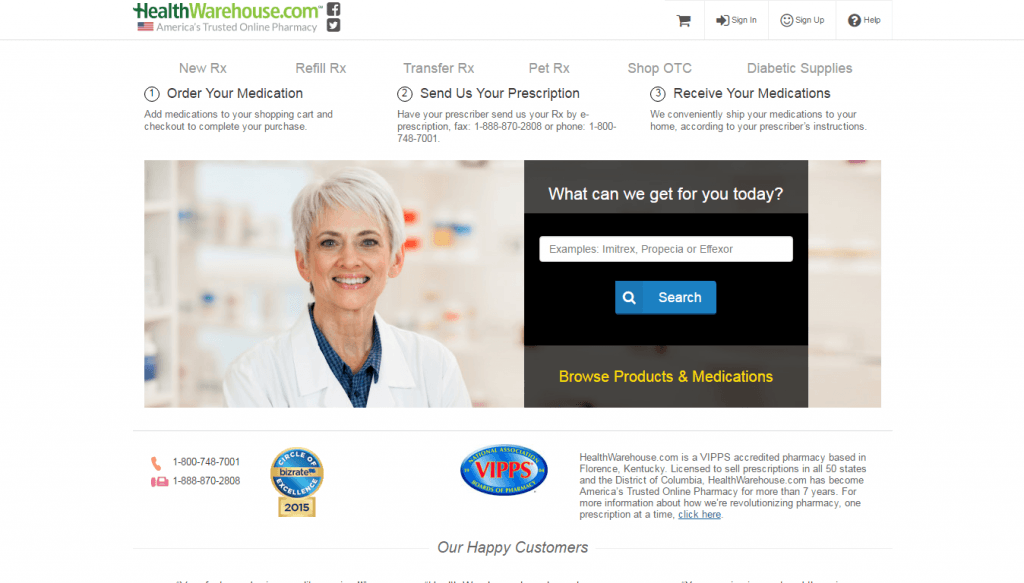**Detailed Caption for Healthwarehouse.com Homepage Image:**

The image showcases the homepage of Healthwarehouse.com, branded as "America's Trusted Online Pharmacy." The website header features their logo, with "health" in dark green, "warehouse" in lighter green, and an adjacent American flag icon, reinforcing the tagline beneath— "America's Trusted Online Pharmacy." 

To the right of the logo are social media icons for Facebook and Twitter. Further right, in the top corner, are icons for a shopping cart, a sign-up section represented by a smiley face, and a help option shown as a black paddle with a white question mark.

Directly below the header menu, a series of service options are displayed: "New Prescription," "New Rx," "Refill Rx," "Transfer Rx," "Pet Rx," "Shop LTC," and "Diabetic Supplies." These options guide users through three main steps:
1. Order your medication and proceed to checkout.
2. Send a prescription by having your prescriber fax it to 1-888-870-2808 or call 1-800-748-7001.
3. Reserve your medications for convenient home delivery according to prescriber directions.

On the left side, a white female pharmacist with white hair and a blue shirt under her lab coat is smiling, adding a personal touch to the page.

A central search bar invites users with the prompt, "What can we get for you today?" followed by example medications like "Imitrex," "Profesca," or "Elixir." Below the search bar, in gray and black, and yellow text it says, "Browse product and medications."

In the bottom left corner, contact information is clearly displayed: 1-800-748-7001 and 1-888-870-2008. Adjacent to this are two award icons: one is a gold circle indicating "Circle of Excellent Service 2015," and the other a gold VIPPS insignia, certifying Healthwarehouse.com as a VIPPS accredited pharmacy.

The company is described as being based in Florence, Kentucky, licensed to sell prescriptions across all 50 states and the District of Columbia. They've earned their reputation by revolutionizing and modernizing pharmacy services, aiming to be America’s top trusted online pharmacy. A call-to-action button reading "Click here" suggests further engagement with the site.